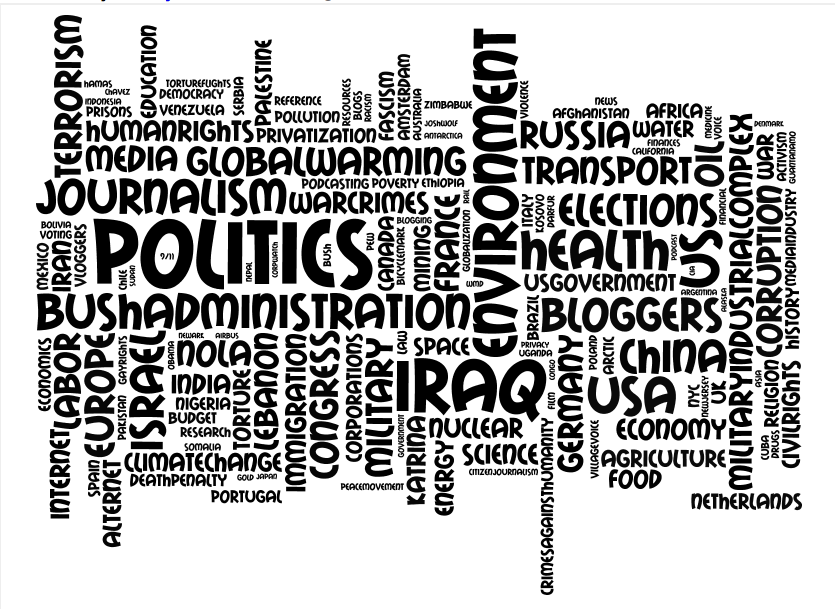The black and white image features a landscape-oriented rectangle background with numerous words in varying sizes. Enclosed by a thin gray border along the top and left edges, the bottom and right sides remain open. The words—all in black font against a white background—are arranged both horizontally and vertically, creating a dynamic, multi-directional layout. The text includes significant terms such as "politics," "Iraq," "health," "USA," "economy," "elections," "Russia," "global warming," "racism," "media," "transport," "China," "Bush administration," "internet," "labor," "terrorism," "environment," "industrial complex," "corruption," "civil rights," "Congress," "Palestine," and "education." Larger bold words such as "global warming," "media," "politics," and "human rights" stand out among other various socio-political themes, capturing a snapshot of contemporary global issues.